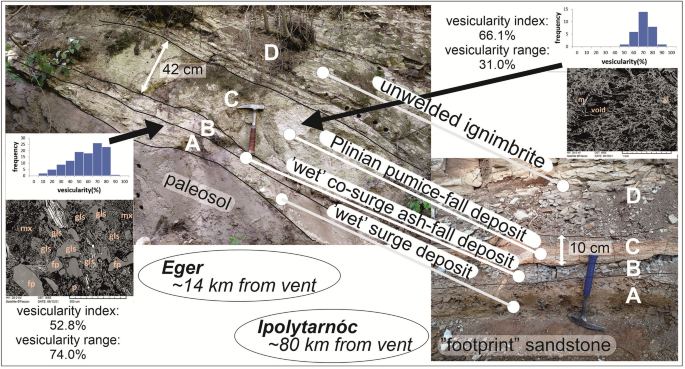This is a detailed overhead color photograph displaying a patch of dry, cracked ground interspersed with weeds, likely from an excavation or archaeological dig site. The terrain is depicted in earthy browns, with metal-gray, blue, black, and white tones highlighting various elements. The image is annotated with extensive text boxes and arrows, which use very technical language to explain the scene. White letters "A, B, C, D" mark specific points of interest. Key terms include "vascularity index" (52.8%) and "vascularity range" (74.0%), "unwelded ignimbrite," and deposits like "pinion pumice fall" and "wet surge ash." Distances such as 14 kilometers to "igur" and 80 kilometers to "Ipolytarnoc" are noted. Two bar graphs, located in the top right and middle left, provide additional data. Hand tools are placed within the photo for scale, illustrating the overall barren and rugged texture of the landscape.